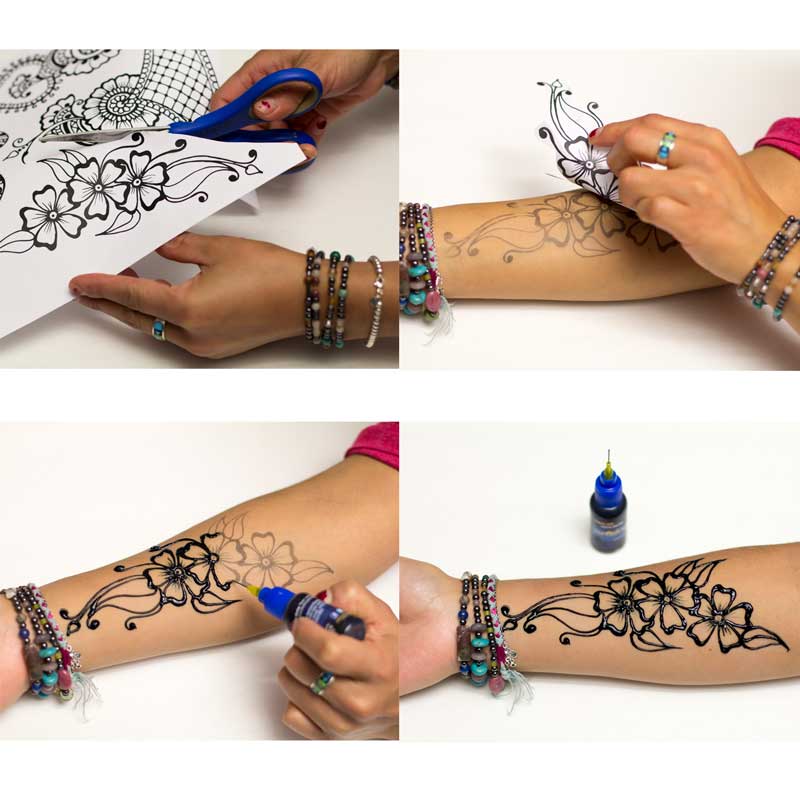The series of four images documents the detailed process of a woman applying a floral tattoo to her arm, possibly using henna or a temporary tattoo technique. In the upper left photo, she is seen wearing numerous ethnic-looking wooden bead bracelets as she uses blue-handled scissors to meticulously cut out a black and white floral design from a piece of paper. The upper right image captures her attaching the cut-out stencil to her arm, transferring the design onto her skin with ink. In the bottom left photo, she traces and fills in the stamped design using a black paint or ink tube, visibly showing part of her pink sleeve and rings on her fingers. The final image on the bottom right reveals the completed tattoo, an intricately outlined floral pattern with leaves, on her arm adorned with the same bracelets against a stark white background. This series collectively illustrates each step of the tattoo application process.